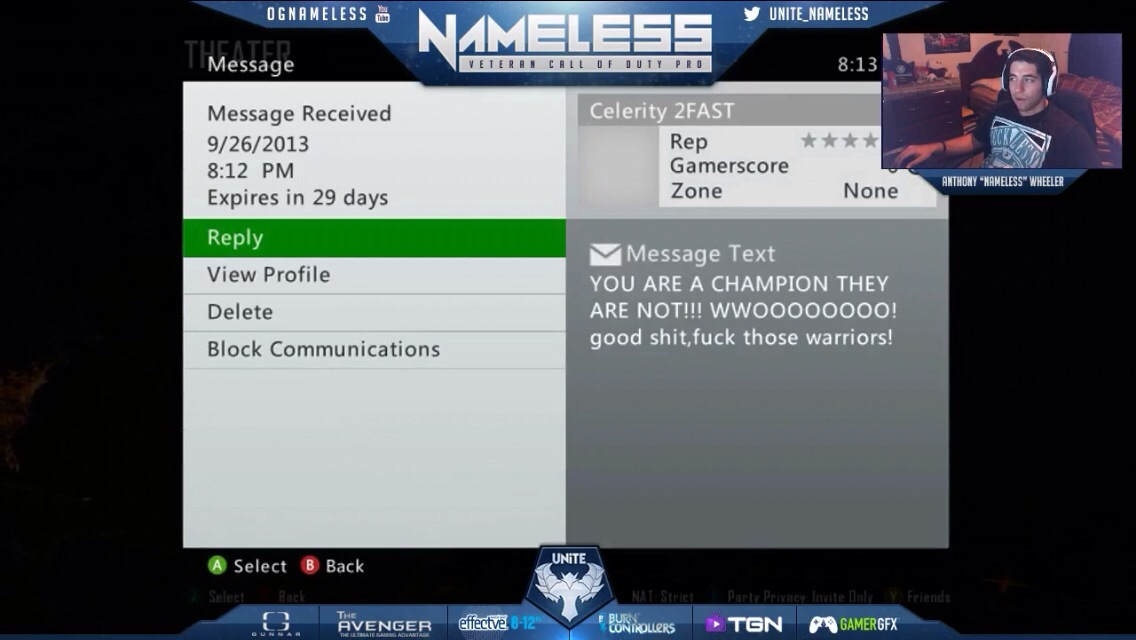This is a detailed screenshot from a live gaming stream featuring Anthony "nameless" Wheeler, a veteran Call of Duty professional player. The main screen displays a message received on 9/26/2013 at 8:12 PM from a user named celerity2fast, reading, "You're a champion they are not woo good shit fuck those warriors." This message, accompanied by options such as reply, view profile, and block communications, is set against a white background on a gray interface. At the top of the screen, "nameless" is written in large white letters on a metallic blue bar, underscored by "Call of Duty." The image includes a small, picture-in-picture box at the top right corner showing Anthony Wheeler, who has medium tan skin and dark hair, wearing white headphones and a black T-shirt with "Reckless" in white font over a green background. In his background, an ornate headboard and dresser are visible, indicating that he is streaming from his bedroom. Above his screen image, "UNITE_nameless" appears, suggesting a team affiliation, and the messages appear in gray on a white background with a green reply bar below. Additional gaming icons and text such as "Avenger," "effective," "TGN," and "gamer SFX" are present at the bottom of the screen, confirming the competitive and interactive nature of the stream.